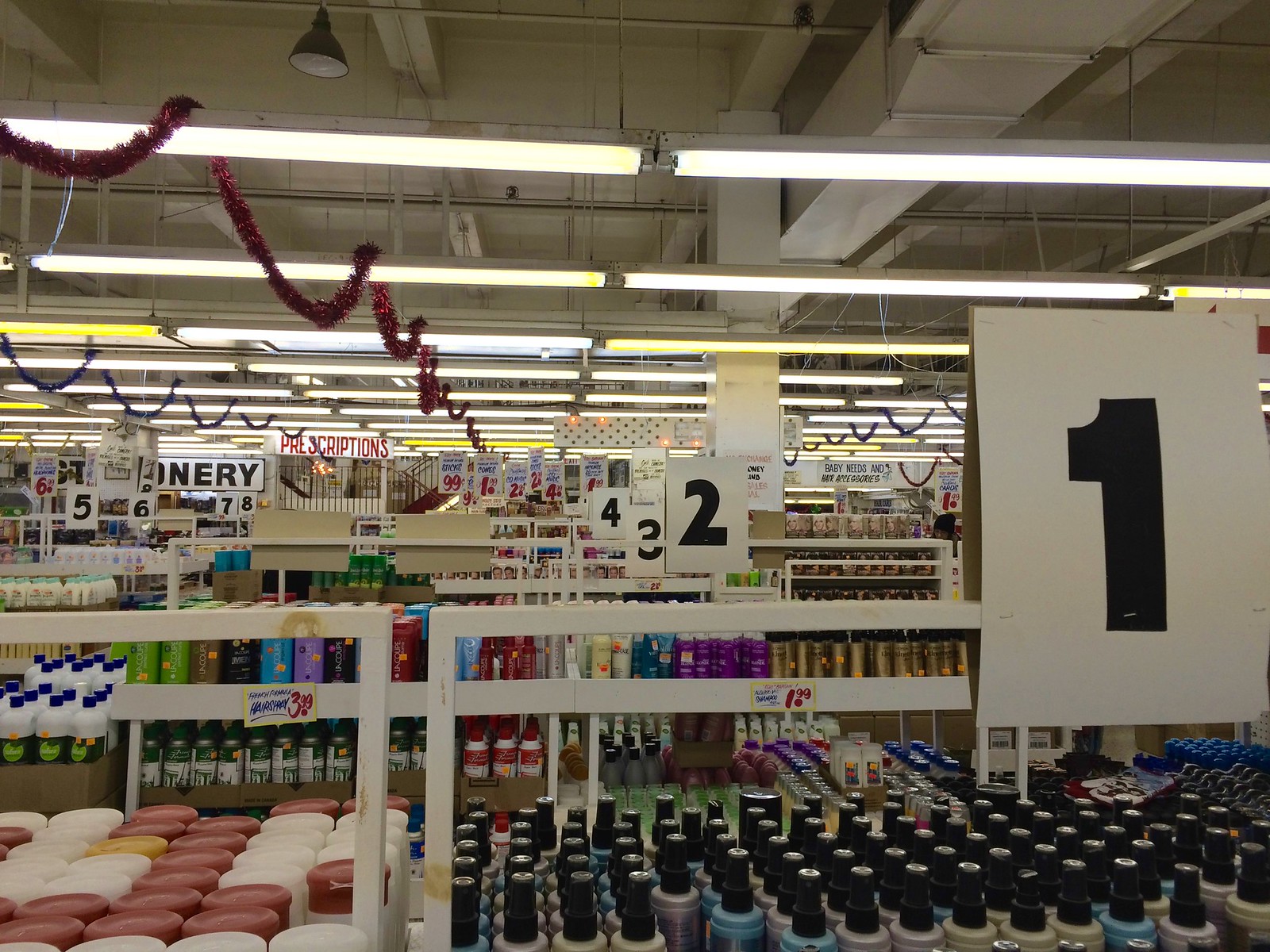The image depicts the interior of a supermarket with a warehouse-like ambience, featuring aisles loaded with a variety of products. Overhead, long, hanging fluorescent lights illuminate the scene, adorned with red Christmas tinsel. The ceiling is exposed, revealing rafters, piping, and venting. The aisles are sequentially numbered with large white signs displaying black numbers from 1 through 8. 

In the foreground, Aisle 1 showcases an assortment of bottles in various colors including blue, green, and brown, some with black caps. To the left, there are additional bottles with either brown or white caps marked at $3.99, and what appears to be nail polish with black caps, possibly OPI, priced at $1.99—a noted bargain. A big sign partially visible on the left spells out "-NERY," and at the very back, a white and red sign indicates the prescriptions section, suggesting the pharmacy might be closed with its barred appearance.

Aisle 2 appears to be part of a hygiene section, lined with numerous colored bottles—likely shampoos—in shades of green, red, yellow, purple, and gold. The entire scene is replete with sales signage, price tags, and advertisements, reflecting a bustling grocery store warehouse filled with a range of products available for purchase.